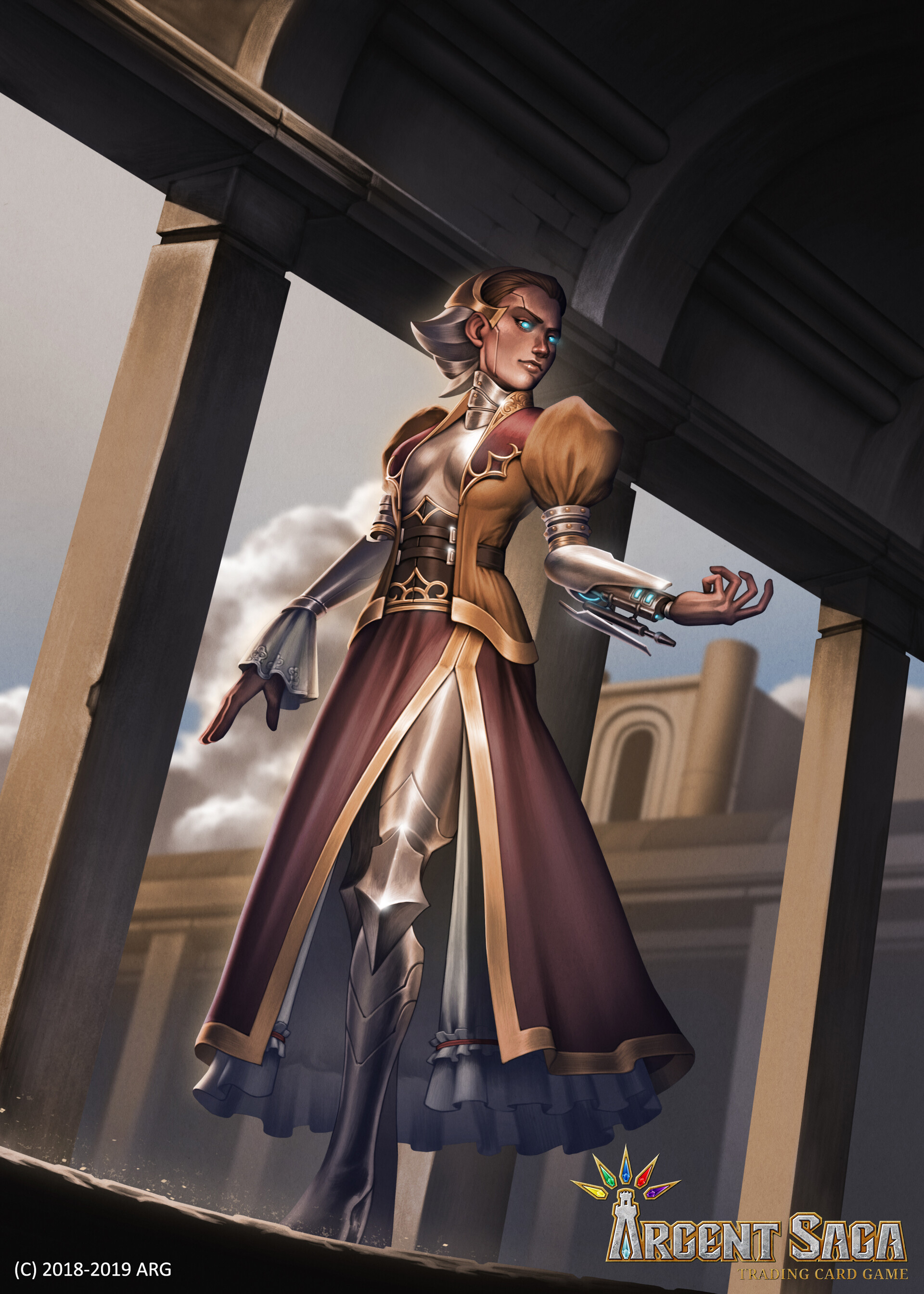The image portrays a highly detailed, animated depiction of a sci-fi inspired woman who appears to be part-human, part-robot. She has distinct brown hair on the top of her head which transitions into metallic components and silver hair below. Positioned in a semi-profile, her striking blue, glowing eyes capture attention. She's adorned in an elaborate outfit featuring a silver neck piece extending to silver elements in the chest area, highlighted by a jacket with golden trim and red accents on the shoulders. The jacket itself is gold outlined with a lighter shade of gold and puffed shoulders. 

Her left arm is extended outward with fingers curled, displaying mechanical intricacies and blue lights alongside elements resembling an arrow and lightning bolt. Her attire includes a prominent brown belt, cinched through the jacket and culminating in a pointed top, paired with a purplish skirt with a blue interior, revealing her metallic legs. She wears high-heeled, knee-length black boots.

The scene is set against a backdrop depicting a cloudy sky and a building, with the woman standing on a structure resembling a wall on a bridge, under a black covering. In the bottom right-hand corner of the image, the text reads "Argent Saga, 2018 to 2019" with additional, less legible text beneath. This artwork powerfully combines futuristic elements with a rich color palette and meticulous design.